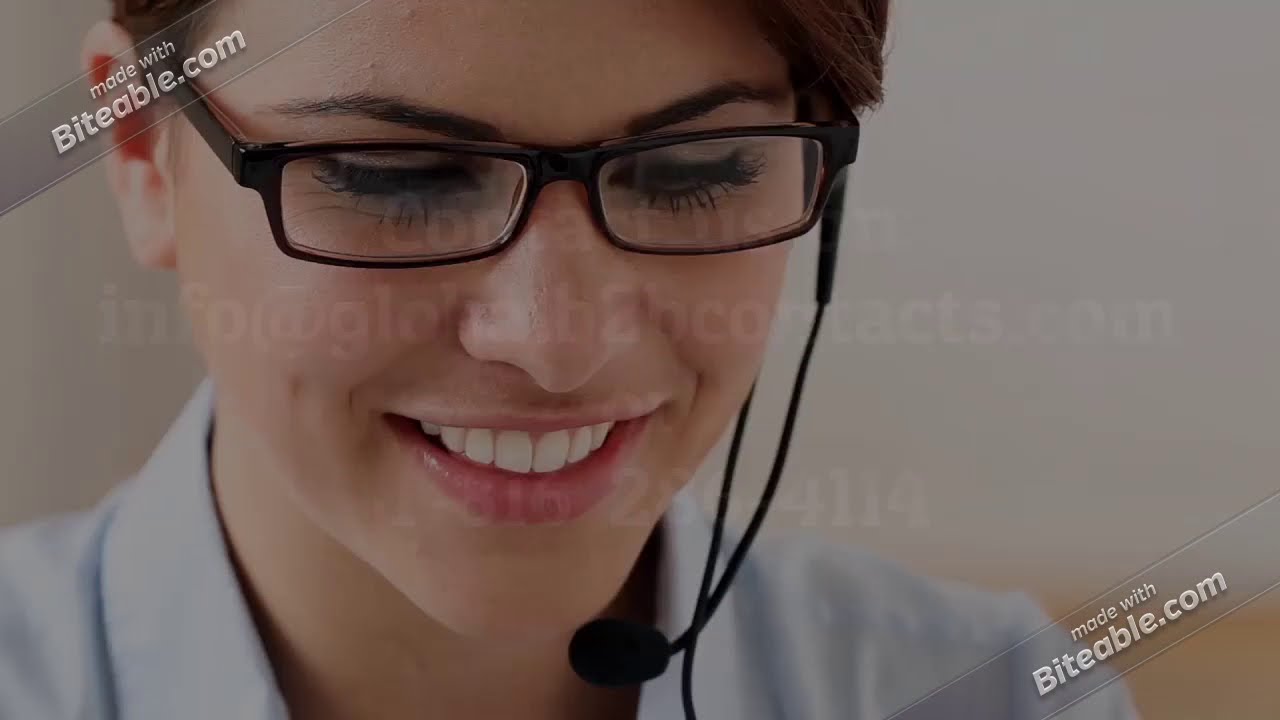The image is a close-up view of a smiling white woman wearing a light blue button-down shirt, indicative of a customer service agent. She has brown hair, and her dark, thin eyebrows highlight her black rectangular prescription glasses with thin frames. Her attractive features include very pink lips and white teeth. She is wearing a microphone headset clipped to her right ear, with a thin wire boom mic fitted with a small foam pad extending towards her mouth. The image is heavily watermarked; oblique, transparent gray rectangles with white text reading "Made with Biteable.com" are present in the top left and bottom right corners. Additionally, faint, nearly unreadable text, including an email address, stretches across the center of the image, contributing to the overall watermarking. The woman appears to be leaning slightly forward, giving the impression of attentiveness typical of a call center representative.